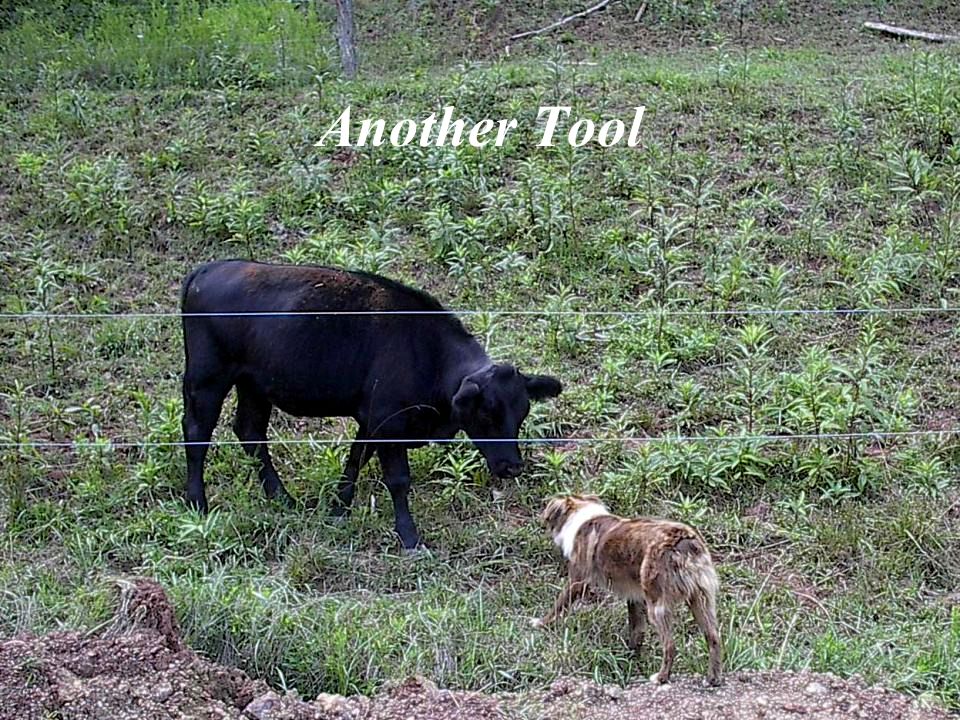In an outdoor scene set against a scrubby field of green and brown grass, a black cow and a brown-and-white border collie face each other from opposite sides of a two-line wire fence that bisects the image horizontally. The ground is a mix of short grass, dirt, and scattered rocks at the very bottom. At the top center of the photo, the text "another tool" is displayed in large white letters. The black cow, positioned above the fence and facing right, bends its head down towards the dog, creating a sense of interaction or curiosity between the two animals. The collie, situated below the fence with its back end towards the lower right corner, looks up at the cow, its left side and back end visible, emphasizing the mutual attention between the pair amidst the rustic landscape.